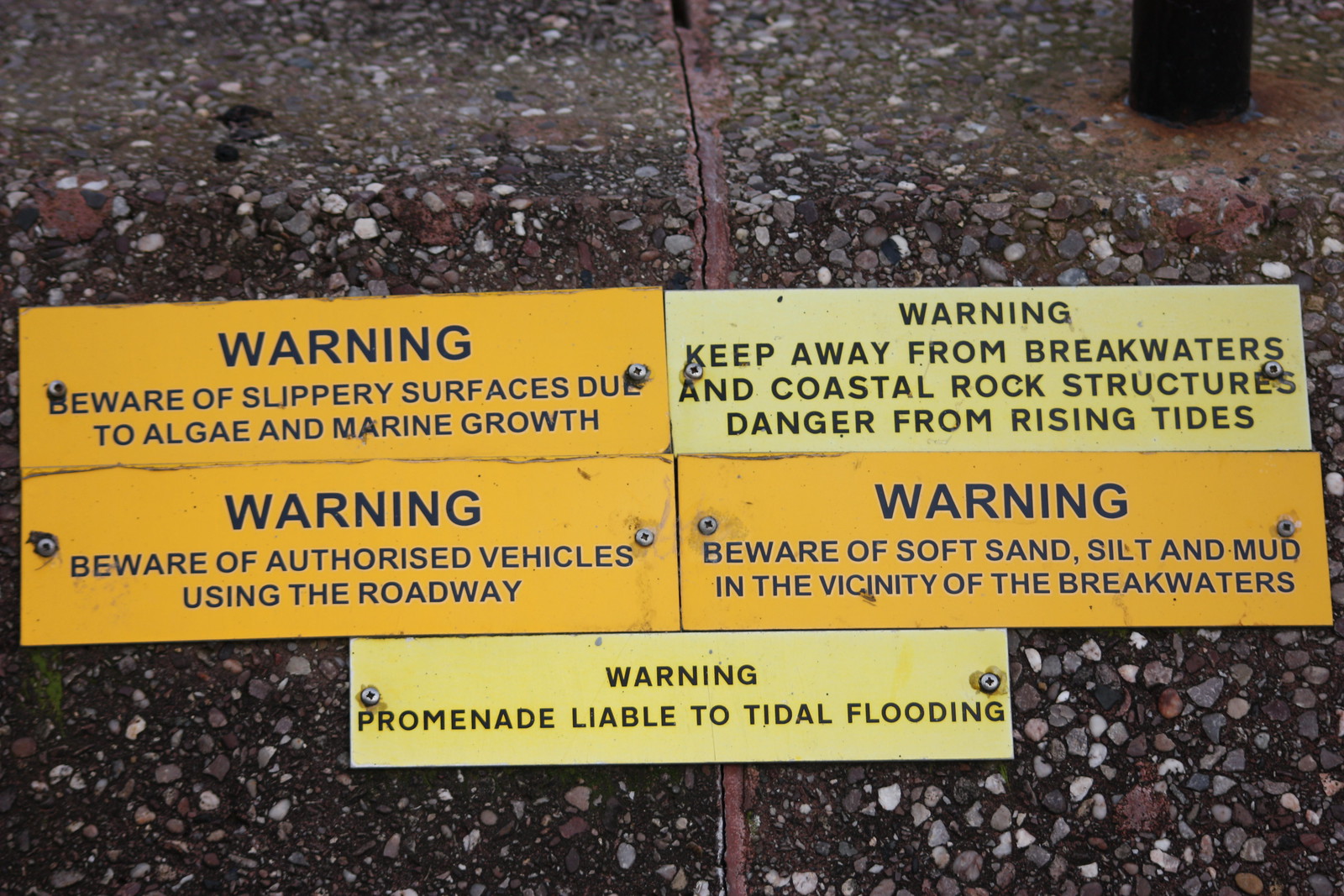The image features a vertical down-view of a cement surface embedded with small pebbles, resembling either a sidewalk or stairs, adorned with five warning signs. At the top of this setup is a small rusted metal post. The background surface exhibits a brown-maroon hue with speckles of grey, white, and pink rocks, adding texture to the scene. These warning signs are meticulously arranged: two on the top row, two on the second row, and a single one centered at the bottom. 

The top-left sign is dark yellow and reads, "WARNING, BEWARE OF SLIPPERY SURFACES DUE TO ALGAE AND MARINE GROWTH" in dark navy text. To its right, a light yellow plaque warns, "WARNING, KEEP AWAY FROM BREAKWATERS AND COASTAL ROCK STRUCTURES. DANGER FROM RISING TIDES," in black font. The second row features another dark yellow sign on the left stating, "WARNING, BEWARE OF AUTHORIZED VEHICLES USING THE ROADWAY" in navy blue. Adjacent to it, also dark yellow with navy text, is "WARNING, BEWARE OF SOFT SAND, SILT, AND MUD IN THE VICINITY OF THE BREAKWATERS." The solitary bottom sign, light yellow with black text, cautions, "WARNING, PROMENADE LIABLE TO TIDAL FLOODING."

Overall, each sign is consistently formatted with "WARNING" in capital letters, indicating various dangers present in this hazardous area.